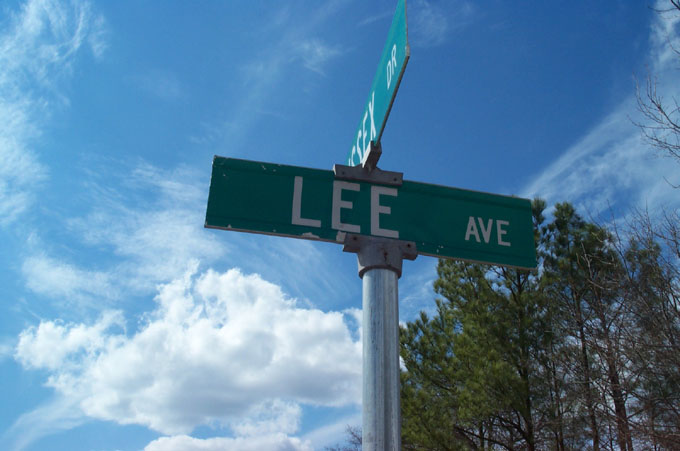In this image, two intersecting street signs form a cross against a vibrant background. The top sign partially reveals the name "Essex Drive," with the characters "SSEX" and "DR" clearly visible. Below it, the sign for "Lee Avenue" is prominently displayed. The photograph is captured from a low-angle perspective, highlighting the uppermost part of the pole that supports the street signs. A clear blue sky dominates the background, accentuated by a large, fluffy cloud situated in the bottom left corner. The scene is framed by the upper branches of a tree, which add a touch of natural detail to the urban setting.